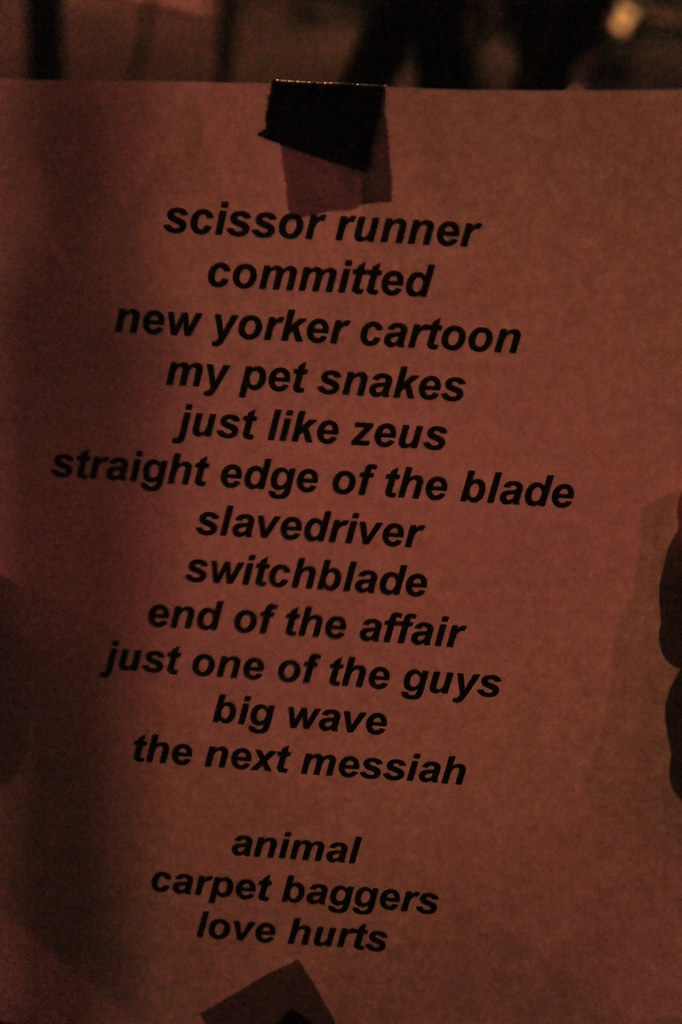This photograph captures a detailed view of a white pamphlet, featuring a list of words or titles printed in black text. The pamphlet includes phrases such as "Scissor Runner," "Committed," "New Yorker Cartoon," "My Pet Snakes," "Just Like Zeus," "Straight Edge of the Blade," "Slave Driver" (repeated twice), "Switchblade," "End of the Affair," "Just One of the Guys," "Big Wave," "The Next Messiah," "Animal," "Carpetbaggers," and "Love Hurts." 

The pamphlet appears to have a black piece of tape affixed at the top, casting a shadow behind it. Additionally, there seems to be another shadow over the bottom middle portion of the tape. A hand, gloved in black, is seen holding the right edge of the pamphlet, contributing to the shadowed effect. The paper displays a small tear or gap on its right-hand side and is slightly tilted to the right.

The overall color palette of the photograph includes shades of tan, beige, brown, and black. The paper itself is described as orangey-browny and appears to be thick. At the bottom of the photograph, a small brown triangle points up to where the words "Love Hurts" are located, adding a final accent to the composition. Despite the thorough detailing, the purpose or context of the list remains unclear.